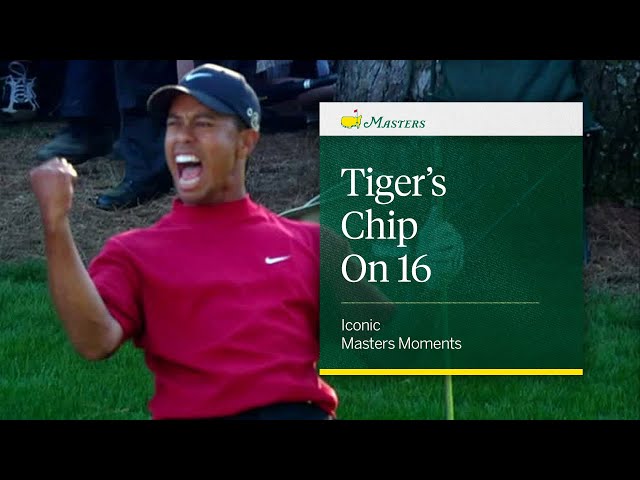This image captures a triumphant moment of the legendary golfer Tiger Woods, celebrating an iconic shot during the Masters Tournament. Focused from his waist to his head and framed with black borders on the top and bottom, the photograph showcases Tiger on his knees, his right fist triumphantly raised. He is wearing a red Nike shirt with the white swoosh logo on his left chest, paired with a black Nike cap. His facial expression is one of elation, mouth wide open mid-yell, eyes squinted in sheer joy. In his left hand, he grips his golf club, which is partially obscured by a green text box on the right side of the image. The text reads, "Tiger's chip on 16. Iconic Masters moments," commemorating his remarkable performance. The background features the legs of spectators standing on a mix of dead grass, dirt, and green course grass, with a tree trunk visible to the right. This appears to be a screen capture from a video clip or a digital slide, highlighting one of Tiger Woods’ unforgettable achievements in golf history.